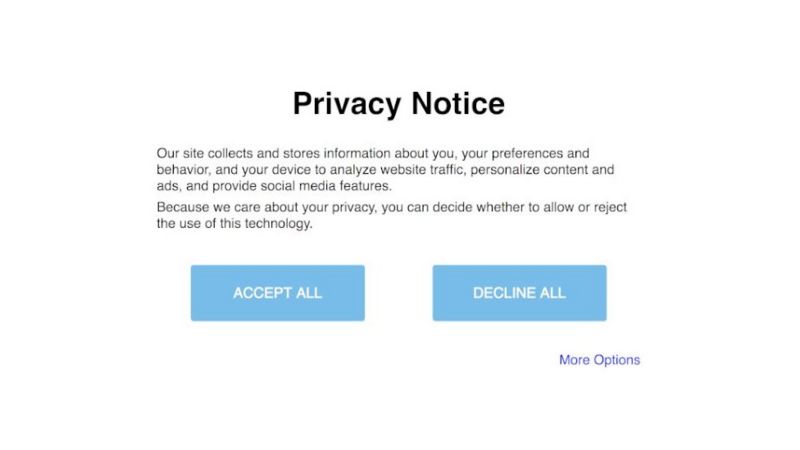The image is a screenshot of a privacy notice displayed on a website. The background is a predominantly off-white color. At the top, "Privacy Notice" is prominently written in bold, black letters. Below this title, there are two paragraphs, also in black text. The first paragraph states: "Our site collects and stores information about you, your preferences and behavior, and your device to analyze website traffic, personalize content and ads, and provide social media features." It continues: "Because we care about your privacy, you can decide whether to allow or reject to use this technology."

At the bottom of the image, there are two rectangular buttons in baby blue. The button on the left-hand side is labeled "ACCEPT ALL" in white, uppercase letters, while the button on the right-hand side is labeled "DECLINE ALL," also in white, uppercase letters. In the bottom left-hand corner of the image, the phrase "MORE OPTIONS" is displayed in blue text.